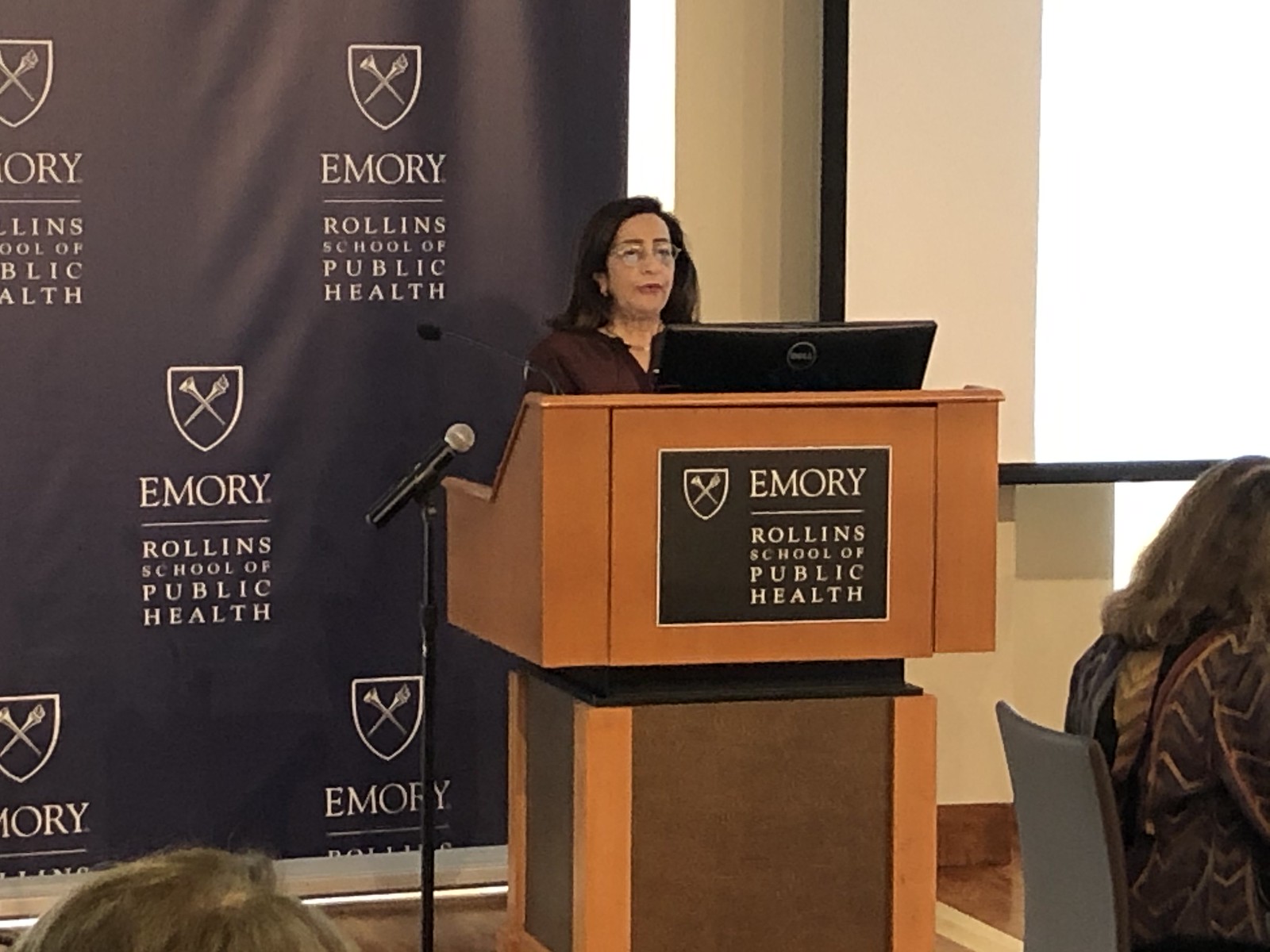The image features a woman with light skin and long brown hair standing at a wide, orange wooden podium adorned with a black rectangle that reads "Emory Rollins School of Public Health" in white font. She appears to be giving a speech, evidenced by her stance behind the podium, in front of a computer screen, and with a microphone positioned to her left. She is attired in a red shirt. The backdrop on the left side of the image is filled with a black screen displaying the "Emory Rollins School of Public Health" logo, which includes a white shield with two crossed objects beneath the word "Emory" and an underline. Behind the speaker, on her right, is a projector screen likely intended for presentations. The setting appears to be indoors during a daytime event, suggested by the visible wooden floor and people seated in chairs, observing the talk.